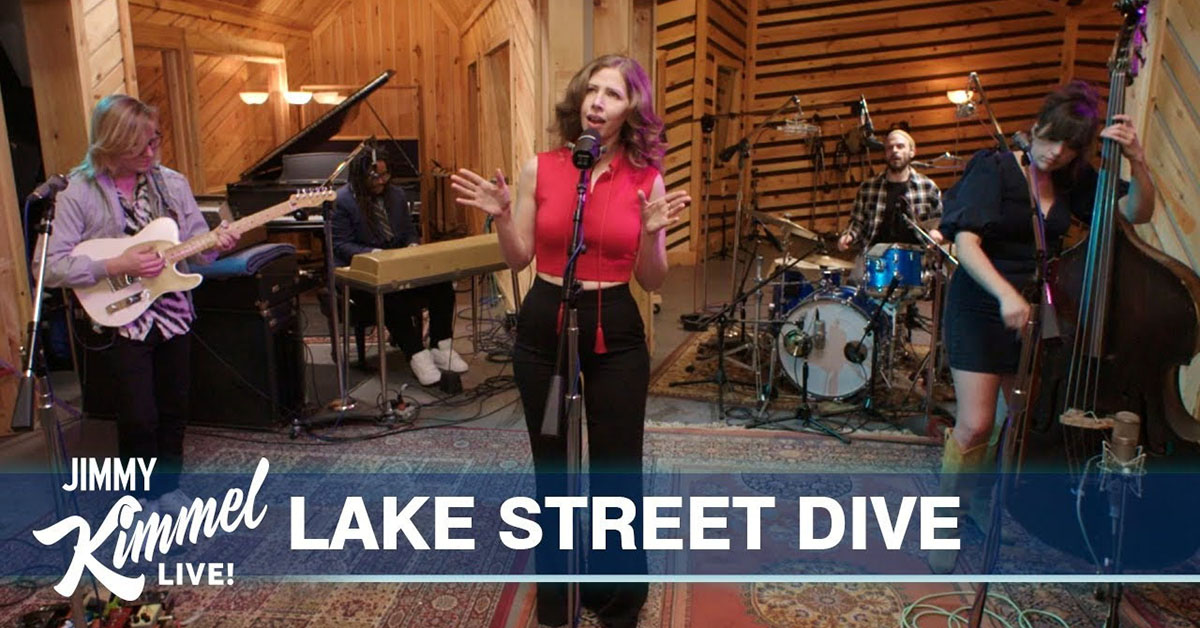The horizontally aligned rectangular image depicts a live performance of the band Lake Street Dive, captured during an episode of Jimmy Kimmel Live. The setting suggests they're playing in a cozy, cabin-like studio with wooden walls and a concrete floor adorned with two large area rugs. At the forefront is the female lead singer, wearing a red crop top with tasseled fringes and black pants, passionately singing with her mouth open and hands outstretched. To the left, a female guitarist in a zebra-patterned shirt, gray jacket, and black pants plays a white guitar. On the right, closer to the back, stands a violinist in front of a drummer, with the latter dressed in a plaid shirt. Also visible in the background on the left is an African American male keyboardist, clad in a dark jacket, striped tie, and white sneakers. Additionally, there's a young female cellist in a black dress and yellow boots. The caption at the bottom of the image features the text “Jimmy Kimmel Live” in white letters on the left and “LAKE STREET DIVE” across the middle.